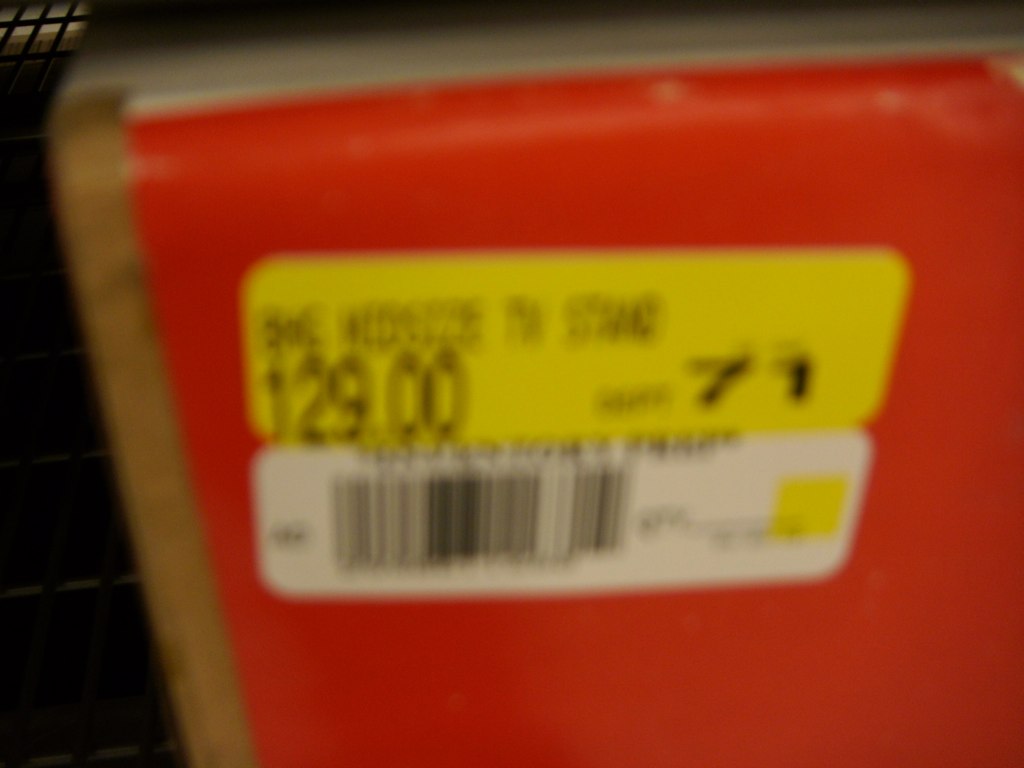The image depicts a blurry price tag affixed to a box, possibly from Best Buy. The price tag displays the cost of $129.00. It is a two-sided sticker positioned over an orange label on the box. The top section of the price tag is yellow, containing the price information, while the bottom portion is white with a small yellow box on the right. The white section includes a UPC barcode, though the text is illegible due to the blurriness.